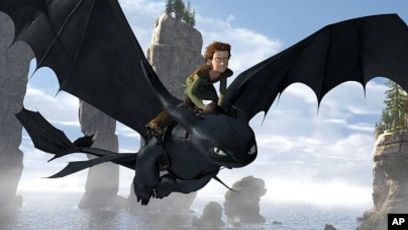In this vibrant frame from an animated movie, a young boy dressed in a Peter Pan-inspired outfit takes center stage, his bright red hair contrasting vividly with his green attire. Mounted on the back of a small, black dragon with bat-like wings, he soars through the sky. The dragon's distinctive long tail ends in a spear-shaped fin, contributing to its fierce yet juvenile appearance. The background showcases tall, imposing rock formations that add a sense of grandeur to the scene. Puffy white clouds dot the bright blue sky, enhancing the whimsical atmosphere. Directly behind the boy and his dragon mount, a towering rocky island composed of brown and gray stones rises majestically. At its peak, four evergreen trees stand tall, adding a touch of greenery to the rugged landscape. In the bottom right corner of the frame, the letters "A-P" are enclosed within a black square, possibly denoting an artistic or production-related mark.